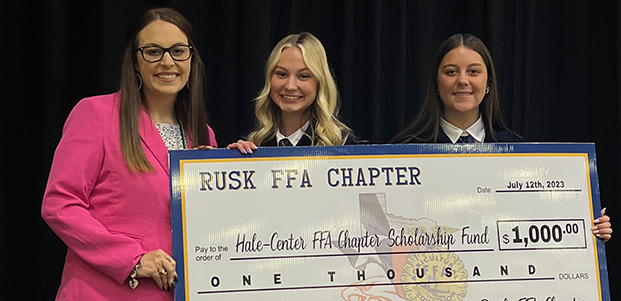In this landscape-oriented, color photograph, three women are standing side by side, smiling at the camera, and holding a substantial replica of a donation check. The check reads "Rusk FFA Chapter July 12, 2023 Hale Center FFA Chapter Scholarship Fund $1,000," with the amount also spelled out in words. The check is light gray with a dark blue border, and inside that, a gold border. The text is in black script, and the check features an illustration of the state of Texas with the state seal.

Starting from the left, the first woman appears to be in her late 30s or early 40s. She has long brown hair parted in the middle, wears black glasses, a pink blazer, hoop earrings, a ring, and a large gold bracelet. The center woman is younger, likely in her early 20s, with blonde hair. She is dressed in a black jacket over a white shirt and tie, resembling a school uniform. To the right stands another young woman of about the same age, with long brunette hair, also wearing a similar black jacket, white shirt, and tie. 

Their hands are positioned on the large check, symbolizing a donation or award, with the backdrop being a dark or black setting that highlights the subjects' bright attire. The scene is suggestive of a formal event or ceremony, possibly related to the Future Farmers of America (FFA) organization.